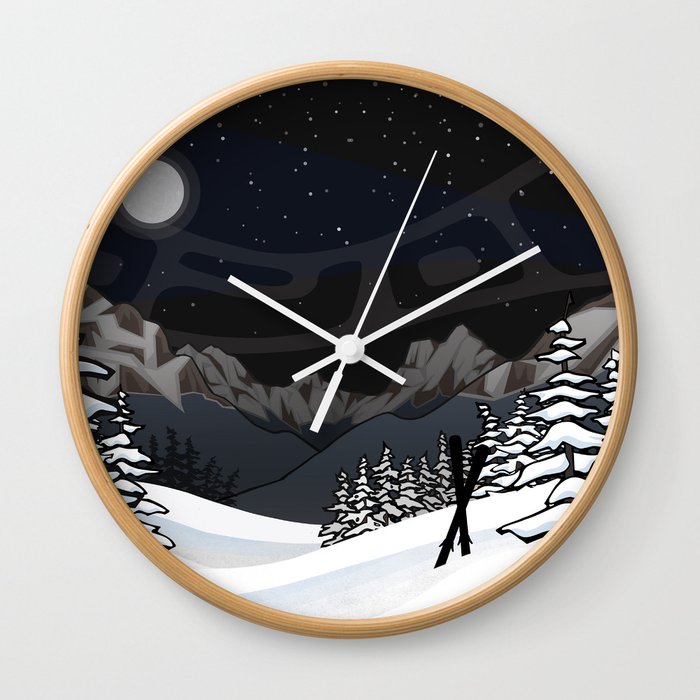This photograph captures a circular wall clock with a plain wooden frame, intricately detailed with an artistic, wintry design in place of traditional clock numerals. The clock face, devoid of numbers, showcases an illustration of a serene snowy scene under a starry night sky. A full moon illuminates the rocky mountain range below, with grey hills cascading beneath them. The landscape eventually transitions into a forest of snow-covered pine or conifer trees, interspersed with snow banks, all rendered in shades of white, black, gray, and tan. The clock is elegantly detailed with white hour, minute, and second hands, all pointing to the time of 10:10:05.